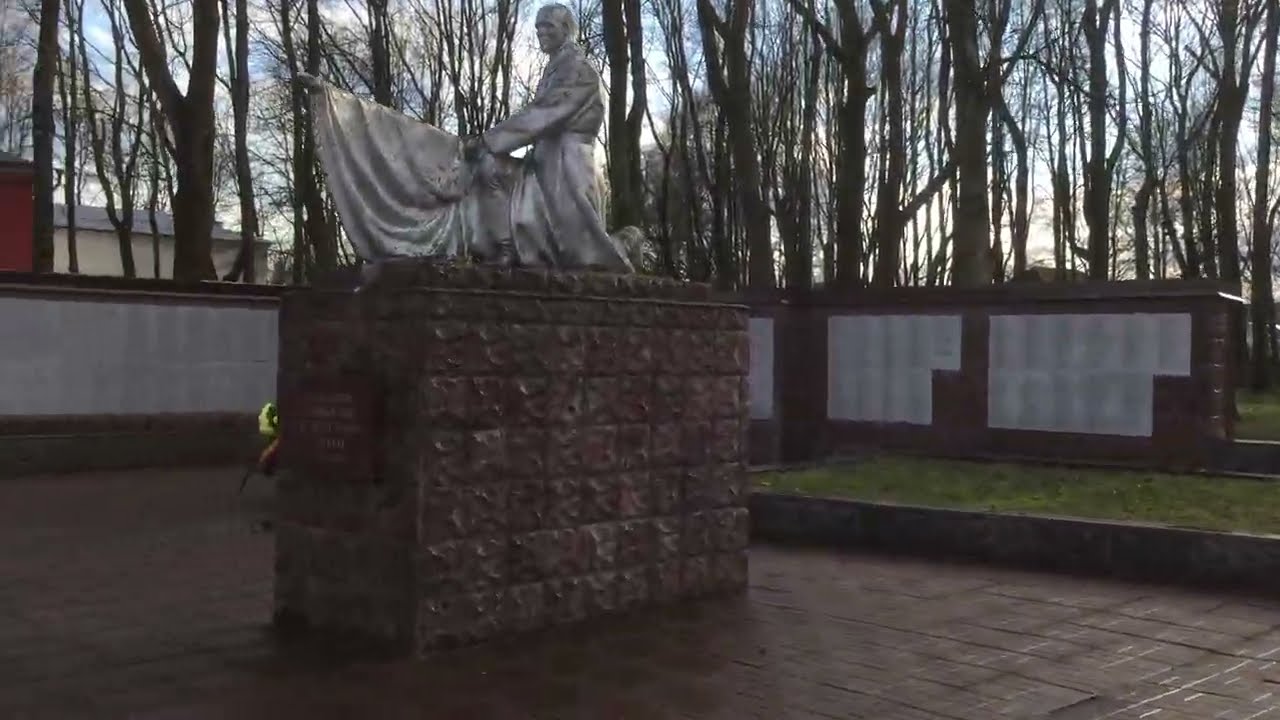The image depicts an outdoor scene featuring a prominent monument. At the center of the scene is a large rectangular platform constructed of decorative brown bricks. Mounted atop this platform is a silver stone statue of an older man dressed in a long coat, holding a long pole with a ribbon or cloth wrapped around it. Surrounding the monument is a brown wall adorned with white pieces of paper, likely containing text, resembling lists of names or places. The scene is further framed by bare trees extending into the distance, indicating that it’s captured during daytime. In the backdrop, there's a mix of green grassy fields and two distinct buildings—one red and the other white with a gray roof. The overall setting includes a raised ledge with grass and a broad, tiled patio below the platform.